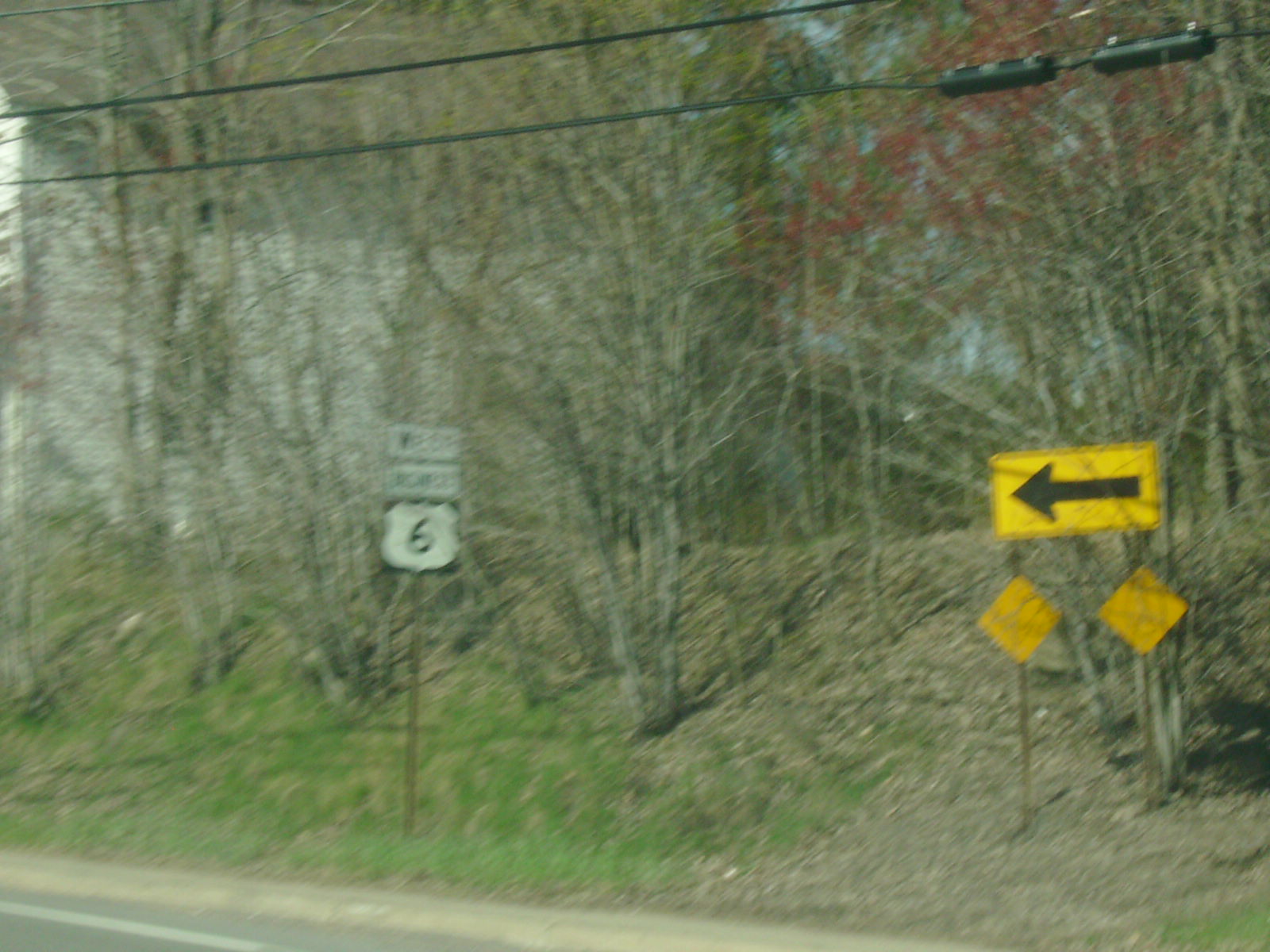This blurred photograph captures the side of a road featuring a mix of natural and man-made elements. Dominating the left side of the image is a portion of the gray street, bordered by a grassy and earthen bank. Atop this bank, there is a prominent yellow road sign with a black arrow pointing to the right, flanked by two smaller reflective yellow diamond signs for enhanced visibility. Nearby stands a Route 6 highway sign, black and white with a large "6" clearly visible, supplemented by two white rectangular signs above it, detailing directions that are not legible due to the image quality. In the background, a sparse woodland of mostly bare trees with a few showing signs of small red flowers, mixed with patches of green grass, creates a forest-like backdrop. Power lines stretch across the top of the scene, possibly leading to traffic signals or electrical infrastructure. A building peeks out amid the trees in the distance, adding to the sense of a rural roadside setting.